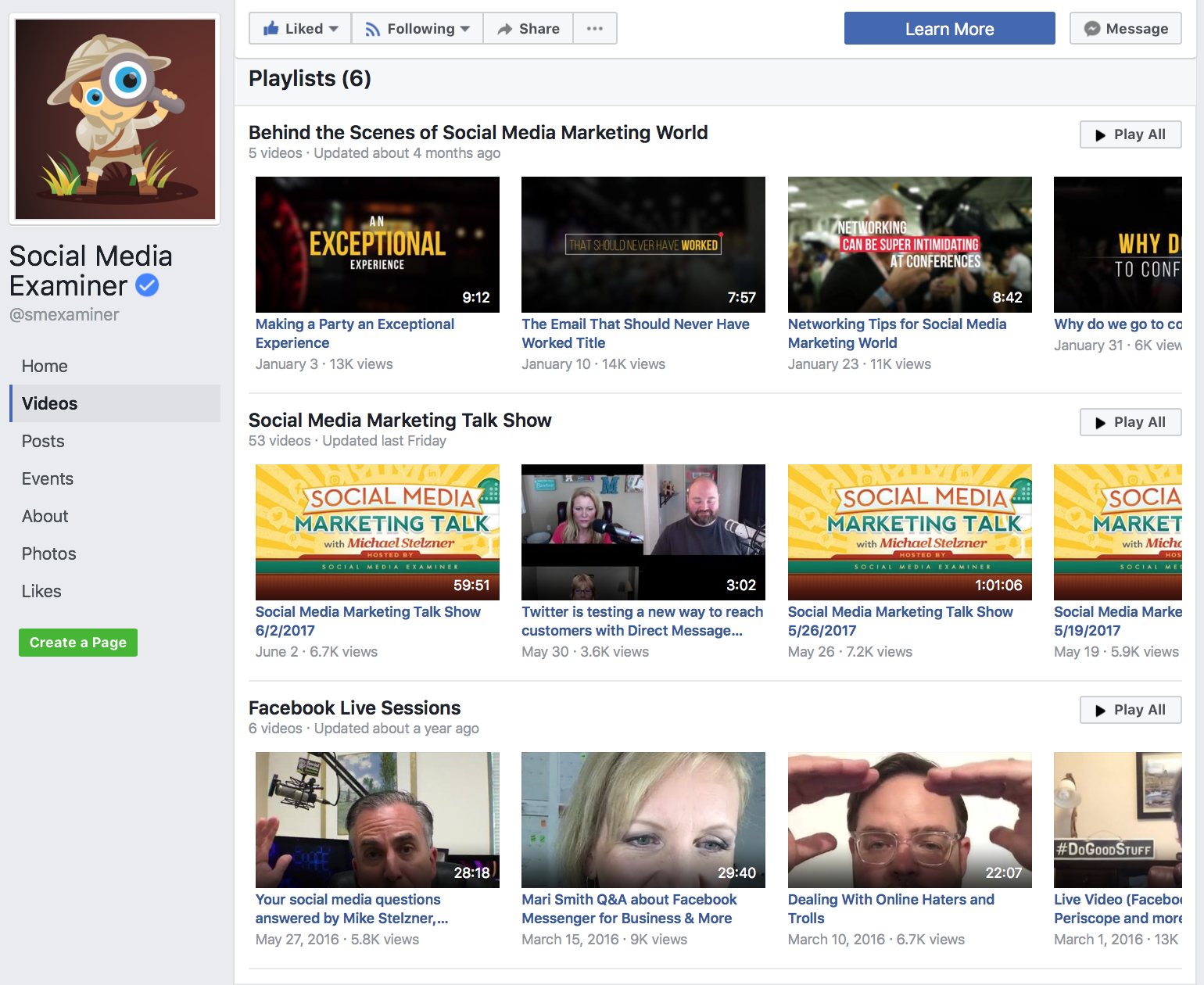This image features a screenshot of a Facebook profile belonging to "Social Media Examiner". The profile photo, located at the top left of the page, showcases a dark red or dark brown background with a cartoon depiction of a man in a safari outfit. The man wears a large magnifying glass over his left eye, which significantly enlarges his blue, circular eye. To the right of the profile picture, the account name "Social Media Examiner" is displayed in black text, accompanied by a verified white check mark within a blue circle.

On the left side of the profile, a vertical menu lists seven tabs in small, black text: Home, Videos, Posts, Events, About, Photos, and Likes. This section sits atop a light gray background.

The main content area on the right side of the screen features a large white background and includes three separate rows, each containing video thumbnails. These thumbnails display either the title pages of the videos or images of people, indicating the availability of various video content and Facebook Live recordings on the profile.